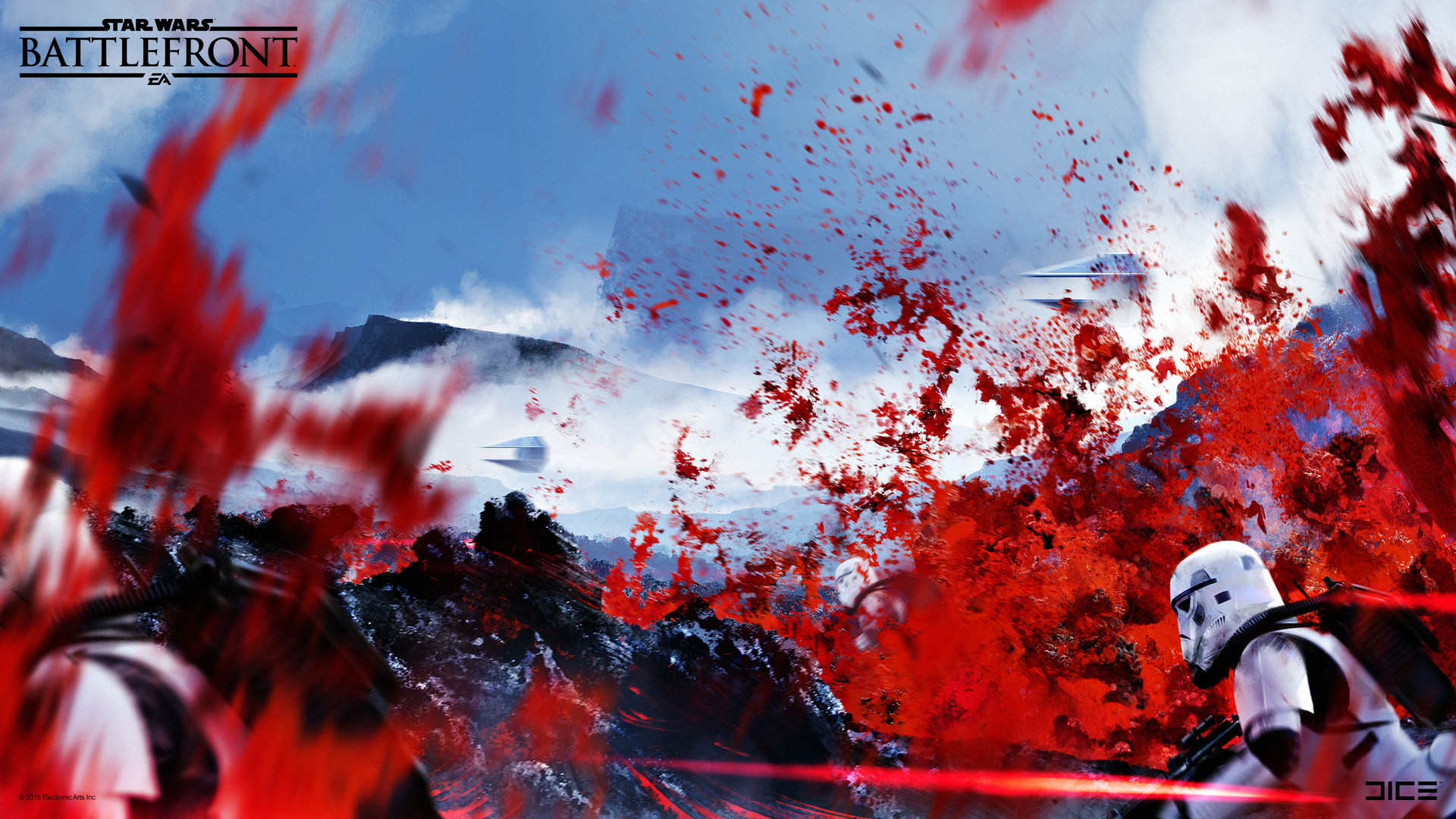In this visually compelling poster for the "Star Wars: Battlefront" video game, the title "Star Wars" is prominently displayed in the upper left-hand corner with the stylish, elongated horizontal lines extending from both S's. Below it, "Battlefront" is framed and highlighted, followed by two additional lines and the EA symbol, denoting the game's publisher, Electronic Arts (EA).

In the lower corner, the word "DICE" is partially obscured, with the left vertical stroke of the D missing, giving it the appearance of a backward C. The background of the poster is dominated by intense red splashes resembling erupting lava amidst a rugged, mountainous, volcanic landscape. On the bottom right-hand side, a detailed depiction of a stormtrooper appears, characterized by their iconic white helmet and uniform. Scattered throughout the stark, black terrain are striking red splashes, enhancing the dramatic effect.

Hovering in the background, several small spacecraft, resembling backwards letter Cs or bird-faced silhouettes, add a sense of dynamic motion and sci-fi ambiance to the scene. This poster effectively combines elements of chaos and heroism, drawing the viewer into the epic battles of the "Star Wars" universe.